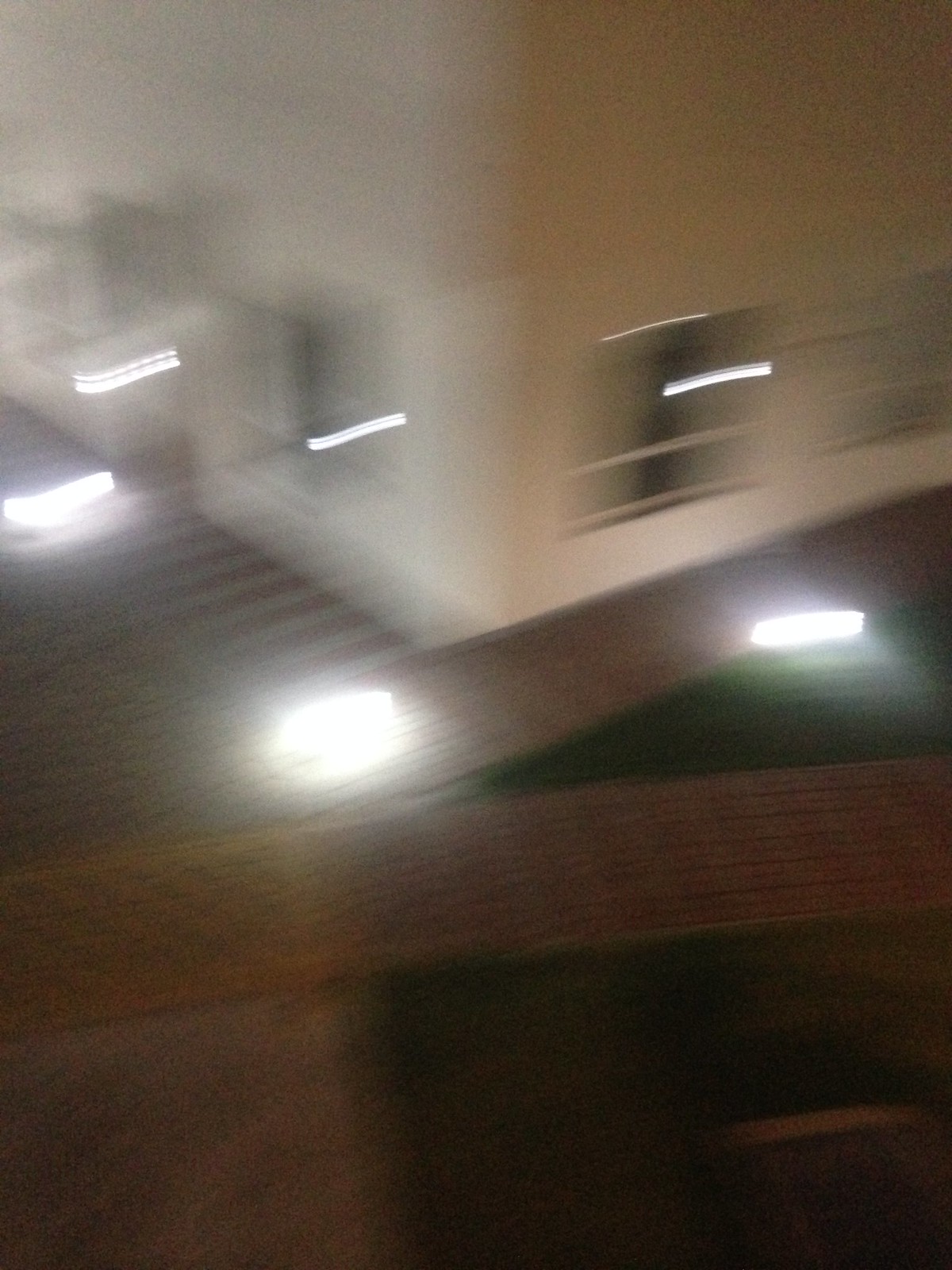A nighttime photograph features a boxy, white building with multiple windows, slightly out of focus. Visible string of bright white lights, spaced roughly 10 feet apart, adorns a ledge just below the windows, illuminating the scene. Below this ledge, the image becomes increasingly blurred, obscuring details. A brown, possibly fabric-like structure resembling an awning is faintly visible, adding a hint of texture to the scene. The lower portion of the image descends into shadow, offering a blend of indistinct black and brown hues.